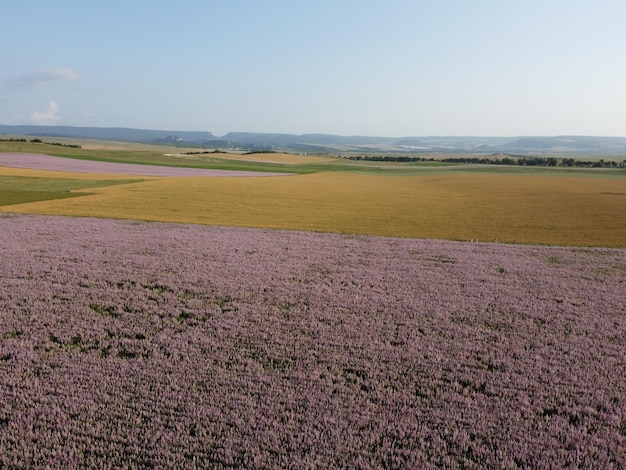This aerial photograph captures a sprawling agricultural landscape marked by vibrant colors and natural beauty. In the foreground, a vast field teems with thousands of purple flowers, possibly lavender, arranged in meticulously planted rows. Adjacent to this is a larger, golden-colored field, likely a recently harvested wheat area, appearing flat and barren in contrast. Amidst the fields, patches of green grass and crops provide additional texture and color. In the top left corner, a small stream meanders through the land, its water shimmering under the pale blue sky. The background reveals a range of purple-gray mountains, gently rolling without sharp peaks, further accentuating the serene setting. Sparse, dusty gray clouds float in the sky, adding to the tranquil atmosphere. Far beyond, the black silhouettes of trees create a natural boundary to this picturesque scene, devoid of human or animal presence, suggesting it may have been captured professionally.